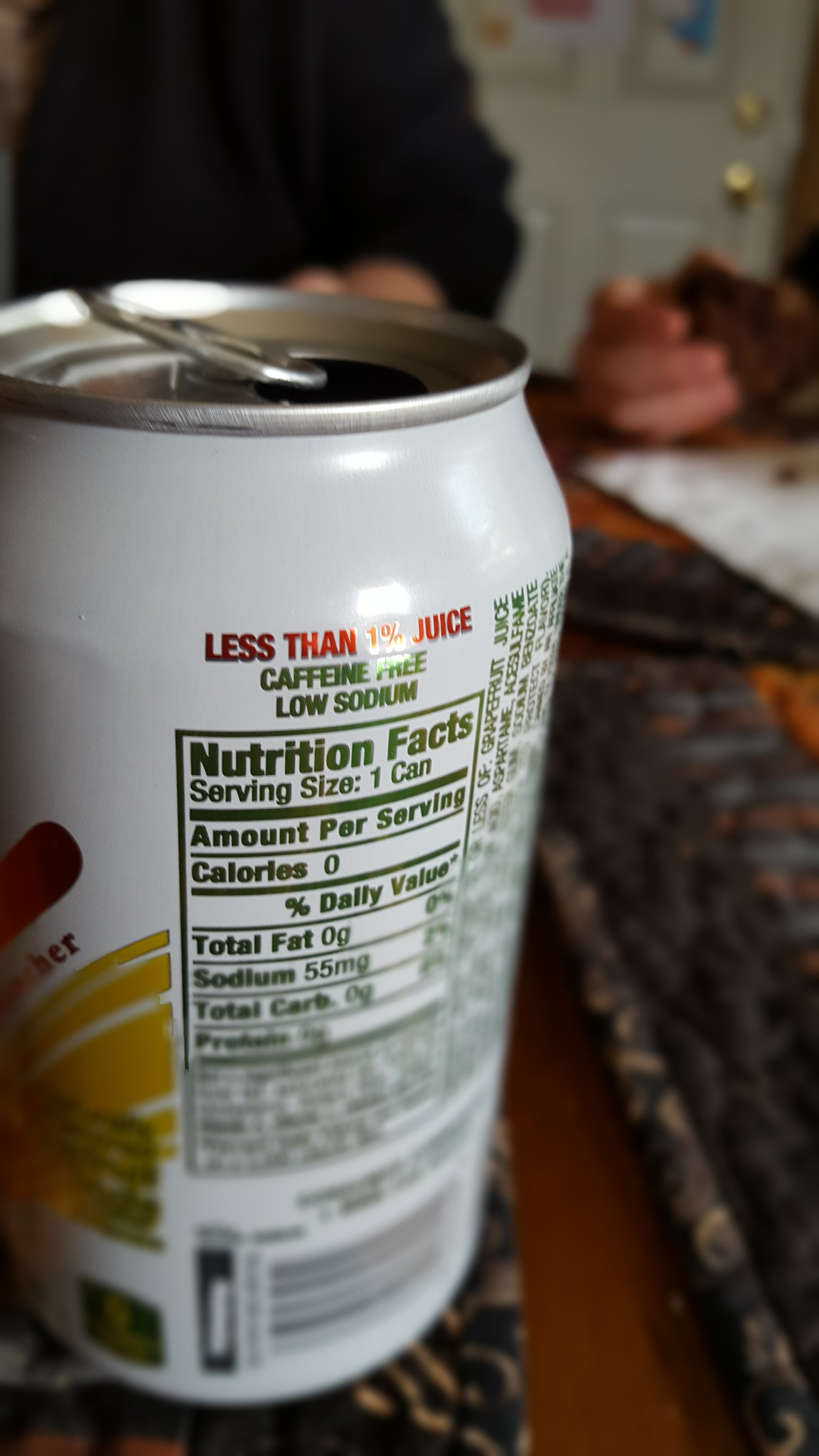A close-up photograph of a 12-ounce, white aluminum can of a caffeinated beverage dominates the left side of the image. The can's nutritional information is prominently displayed, featuring 'Sodium' in green text and a label in red indicating 'Less than 1% juice'. Additionally, the can mentions 'Low sodium' and other caffeine-related information in green. On the right side of the image, there is a partial view of a room, which includes a blue and orange bed and a portion of a white door at the top right. A white hand is visible in the upper right corner near the door. The bottom part of the image shows the front of the can, though the branding and name are blurred and indistinct. The overall scene is set in an indoor environment with a casual, lived-in feel.